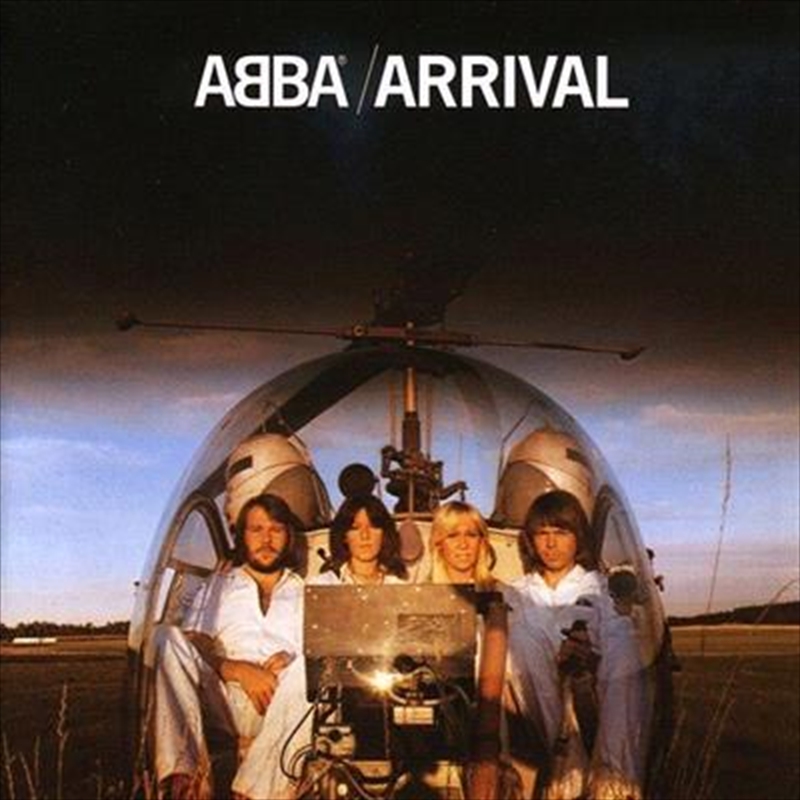The image appears to be an album cover for the band ABBA, formatted in a square shape. At the top of the image, against a solid black background, "ABBA / ARRIVAL" is prominently displayed in all caps with white letters, centered. Notably, the first B in ABBA is backwards.

The main focus of the image is the group ABBA seated inside a large glass, dome-shaped helicopter cockpit, resembling a bubble. Above the cockpit, a rotor blade is visible stretching horizontally across the picture. The scene is set against a backdrop of a light blue sky with white and gray clouds, gradually darkening towards the top, hinting at impending storm clouds.

Inside the cockpit, there are four members of ABBA. On the far left is a man with a brown beard and mustache, short brown hair, and dressed in a white outfit. To his right is a woman with slightly long brown hair, and next to her is another woman with slightly long blonde hair. The man on the far right, also in a white outfit, has shoulder-length brown hair. In front of the women, there appears to be a control panel or monitor, partially obscuring their lower bodies.

The setting appears to be outdoors, with a field, possibly farmland, at the bottom of the image. Some grass blades and twigs are visible in the foreground, and there are trees in the distant background, reinforcing the outdoor atmosphere. The overall composition suggests a promotional image or album cover, capturing a blend of technological and natural elements around the iconic band.